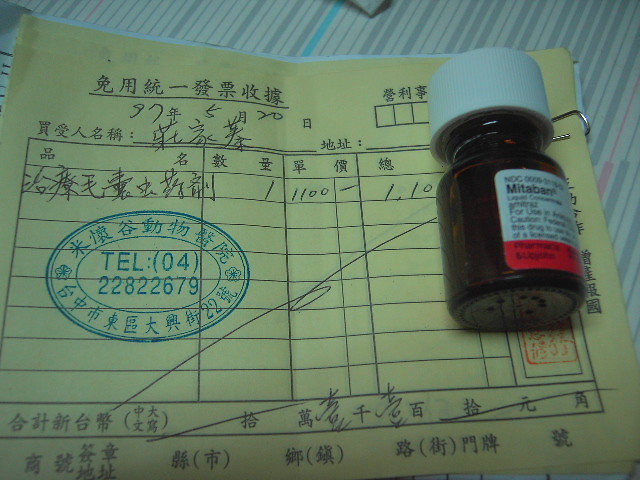The image showcases a detailed top-side diagonal view of a yellow sheet of paper, likely a medication prescription, written entirely in Asian characters, which appear to be either Japanese or Chinese. This yellow paper features a printed chart filled in with these characters, with one line specifically filled out, indicating it might be a form or an official document. A distinct green or blue stamp, resembling a seal, is present on the left side of the paper. Situated on the right side of the paper is a small, dark brown, semi-transparent pill bottle with a white safety cap that requires squeezing to open. The bottle bears a prescription label with bold lettering that reads "Mitaban" or "METABEN." The photograph seems to have been taken in a dimly lit room, adding to the overall subdued and clinical atmosphere of the scene.